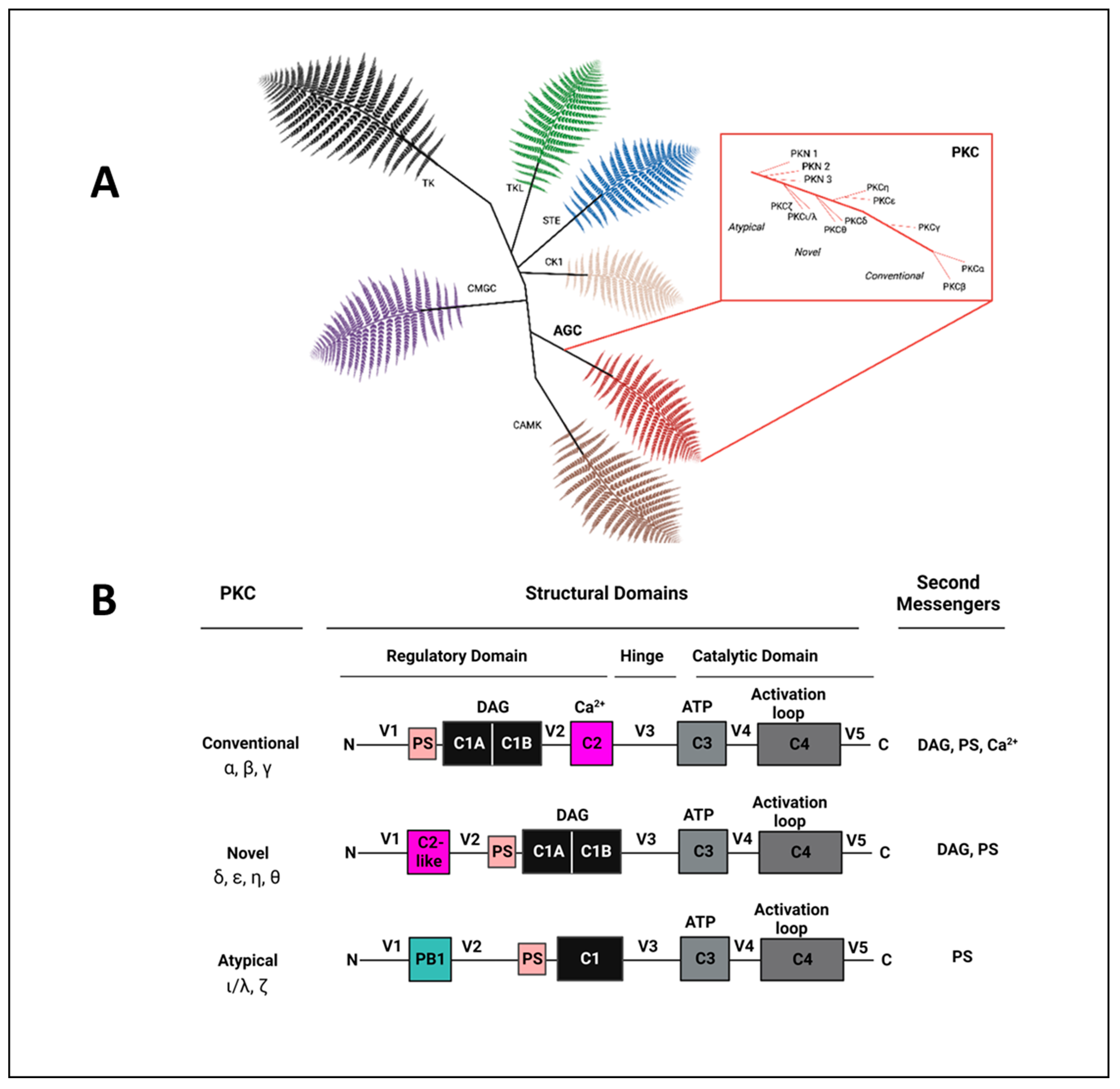The two-part image is a detailed scientific diagram used in chemistry to break down the structural domains and second messengers of protein kinase C (PKC). The top half, labeled "A," features a complex structure that resembles tree branches with fern-like leaves in various colors – black, green, blue, tan, red, brown, and purple – each corresponding to different chemical components and processes. These leaves have labels such as TX (black) and ACE, GC (red). A close-up from the red branch categorizes these components into atypical, novel, and conventional segments, explaining their specific roles. The bottom half, labeled "B," further elaborates on the PKC structural domains, listing elements such as CA1, C1B, ATP, and activation loops alongside second messengers. The entire diagram, devoid of a background, serves as a comprehensive visual aid to outline the chemical composition and functions within the PKC structure.